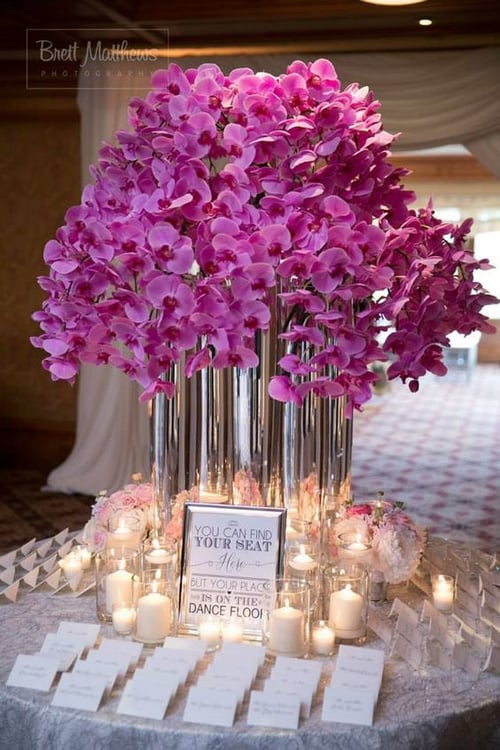A round table draped with a pinkish tablecloth featuring subtle gray streaks is decorated with an array of pink and purple Phalaenopsis orchids in a silver vase that extends upwards and outwards with a mixture of dark and light small petals. At the center of the table is a rectangular sign that reads "You can find your seat here, but your place is on the dance floor," flanked by white candles enclosed in glass cases, casting a warm yellow glow. In front of the sign is a neatly arranged display of place cards, organized in six rows of four cards each, featuring illegible black lettering due to its small size. The background reveals an out-of-focus carpet with a crisscross design of gray lines and light gray centers dotted in the middle. In the upper left corner, blending with the background, is the faintly visible text "Brett Mathers" enclosed in a square, though additional text below it is obscured due to poor contrast.